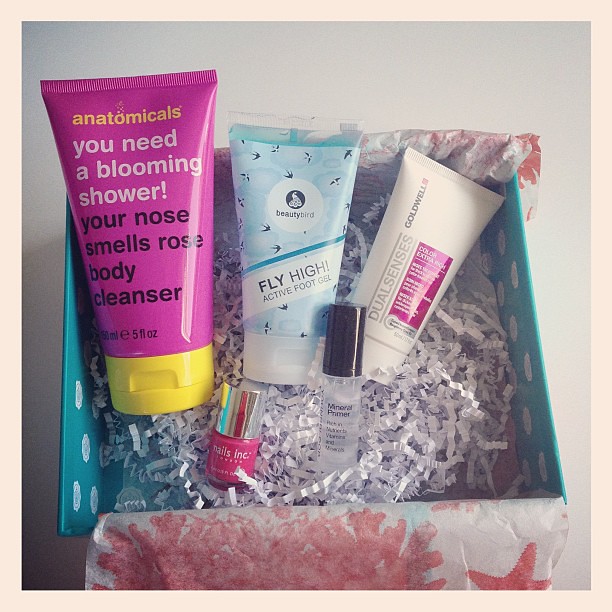The photograph depicts a square gift box, turquoise blue with white dots, resting on a light blue surface. The box is filled with white shredded tissue paper adorned with pink flowers and a pinkish-red star design. Nestled atop the paper are several body care items. Prominently, there is a large bright pink tube with a yellow lid labeled "Anatomicals You Need A Blooming Shower Your Nose Smells Rose Body Cleanser." Adjacent to it is a blue tube with small black bird designs marked "Fly High Active Foot Gel" by Beauty Bird. Another item is a white tube with a magenta rectangle next to the gray text "Dual Senses" by Goldwell, though the remaining text is unclear. Additionally, there is a small bottle of clear liquid labeled "Mineral Primer," purportedly rich in nutrients, vitamins, and minerals, although the text isn't fully readable. Completing the assortment is a pink nail polish bottle with a silver cap, identified as "Nails Inc." The entire image is framed by a light pink border, suggesting this may be a curated gift or a product display.